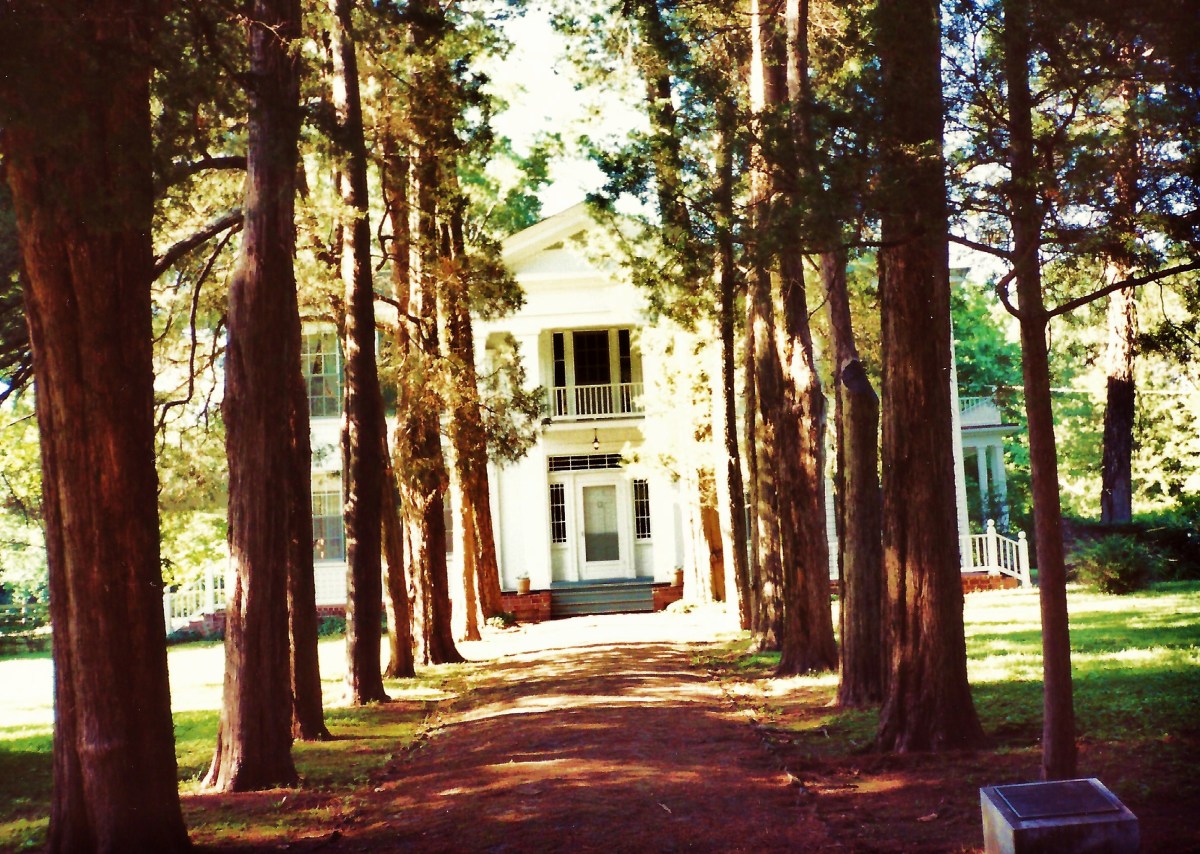The image portrays a serene, sunlit afternoon at a sizable, two-story white plantation home, possibly situated on a farm. A dirt and grass path, bordered by a precise line of rocks, leads up to the stately mansion. This path is flanked by rows of tall, majestic trees with sturdy brown trunks. The house features a prominent balcony above the front door, and an additional side door accompanied by white steps and a railing, visible on the right-hand side. The second story of the home includes a balcony with a small fence gate. The facade of the home is complemented by various windows on both stories and columns that hint at a porch area. The overall scene is devoid of any people, capturing the tranquil beauty of the plantation amidst the expansive surroundings.